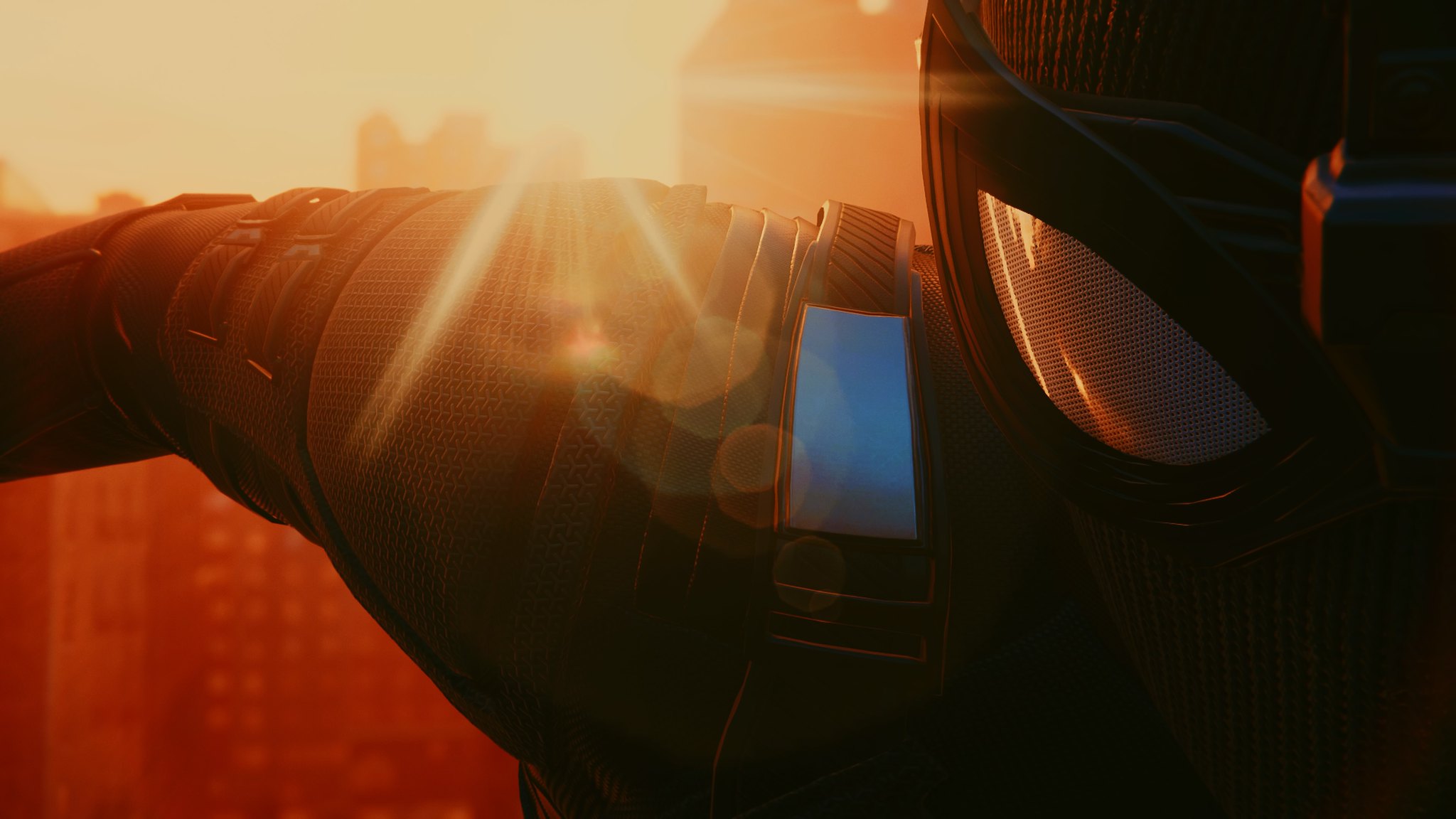The image presents a scene reminiscent of a movie or a video game, featuring a dramatic, bright burst of sunlight that creates a starburst effect in the otherwise dull, grayish sky. The background showcases a silhouette of reddish-hued buildings, which enhances the scene's cinematic atmosphere. In the foreground, the black-suited Spider-Man is partially visible, with detailed focus on an arm, shoulder, and half of his masked face. The distinctive gray mesh eyes and the armored texture of his suit are clearly depicted, exuding a sense of strength and stoic resolve. The mask is fully concealing, leaving no part of the face exposed. A striking blue light on Spider-Man's shoulder stands out, in conjunction with the sunspots that subtly play across his form.